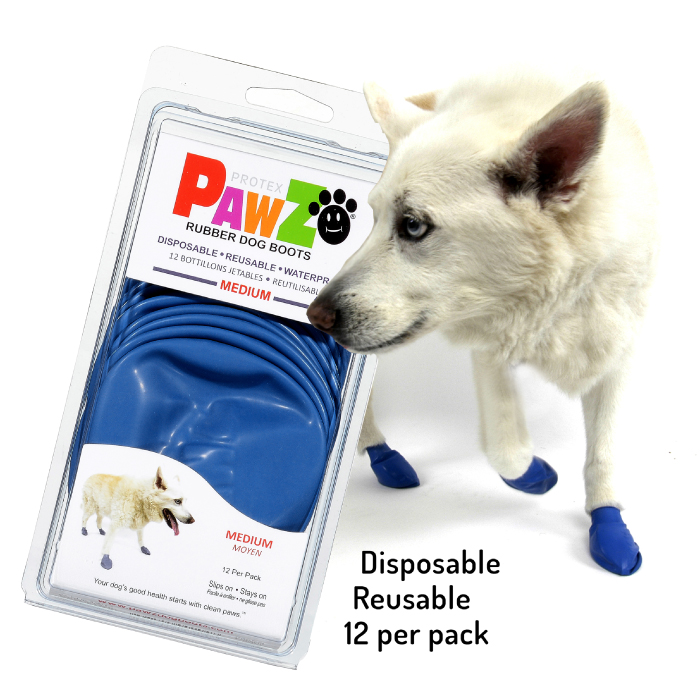This advertisement for Protex Paws Rubber Dog Boots features a detailed collage of images and text. In the upper right, there is a white dog with blue eyes, shown walking towards the viewer while turning slightly to its right. The dog is wearing blue, rubbery booties on three visible feet. Although the dog does not appear very happy in this image, the package on the left side of the collage shows a different picture of the same white dog, who looks happier with the boots on. The packaging, made of clear material, displays multiple blue rubber boots and prominently features branding that reads "Protex Paws," with each letter of "Paws" colored red, pink, orange, and green. The package includes the details: "Disposable, Reusable, Waterproof, Medium, 12 per pack." Additional text over the collage reinforces these attributes, reading "Disposable, Reusable, 12 per pack," and highlights the tagline "Slips on, stays on. Your dog's good health starts with clean paws." The product photo is set against a white background, enhancing the visibility of the items.